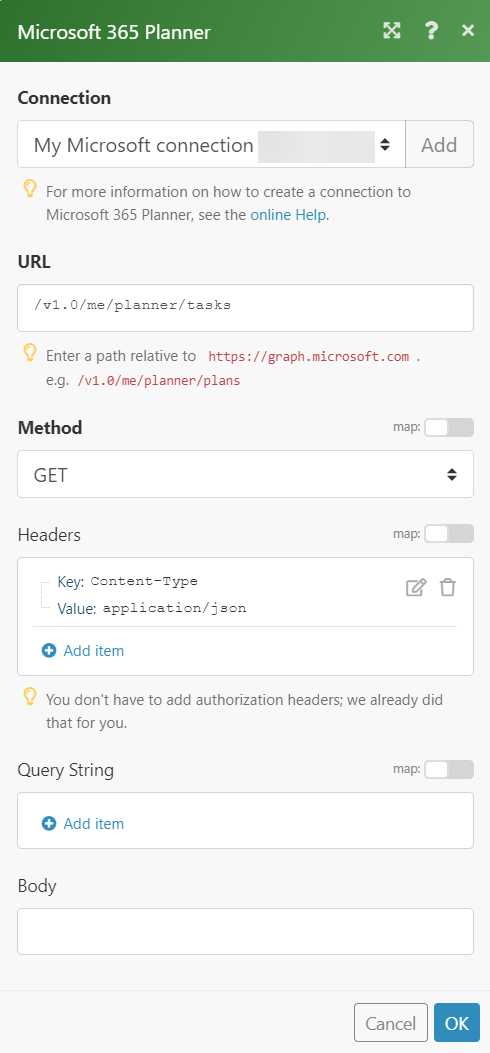This image is a cropped screenshot captured from a mobile device, displaying a web page or a mobile software application. The top of the image features a green rectangular banner with the text "Microsoft 365 Planner." Positioned on the right side of the banner are three icons: one with four arrows pointing outward, a question mark, and an X symbol. Below the banner, the rest of the background is predominantly grey, presenting an input-style form.

The form starts with a section labeled "Connection," featuring a drop-down button and an "Add" button. Below this, there is a text entry field for a URL. Following the URL input, another section labeled "Method" displays a pre-entered "GET" option. Further down, the form includes areas for additional details such as headers, a query string, and a body, suggesting the interface is designed for establishing an authenticated connection between two platforms or services.